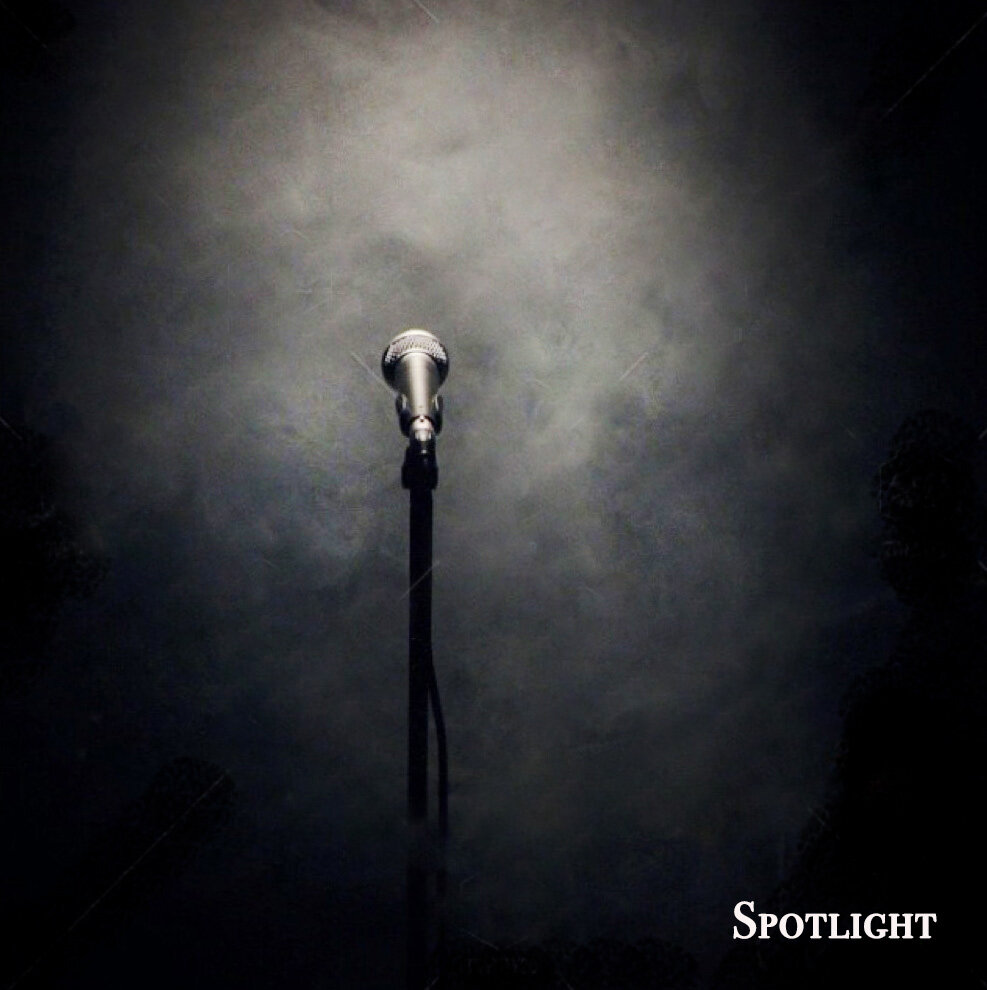The image depicts a dimly lit scene dominated by a black background that fades to a smoky white in the center, transitioning to grayish and purplish hues towards the bottom and right. In the bottom right corner, the word "SPOTLIGHT" is prominently displayed in white capital letters, with the 'S' notably larger than the other letters. Central to the composition is a silver-colored microphone mounted on a black stand, which rises from the bottom of the image. The microphone is oriented away from the viewer, with a visible black holder securing it at the middle of its shaft. A cable is attached mid-way along the stand, extending to the right before descending out of view. The overall atmosphere suggests a stage or performance setup, accentuated by a fog-like texture that catches the light, adding a sense of depth and moodiness to the scene.